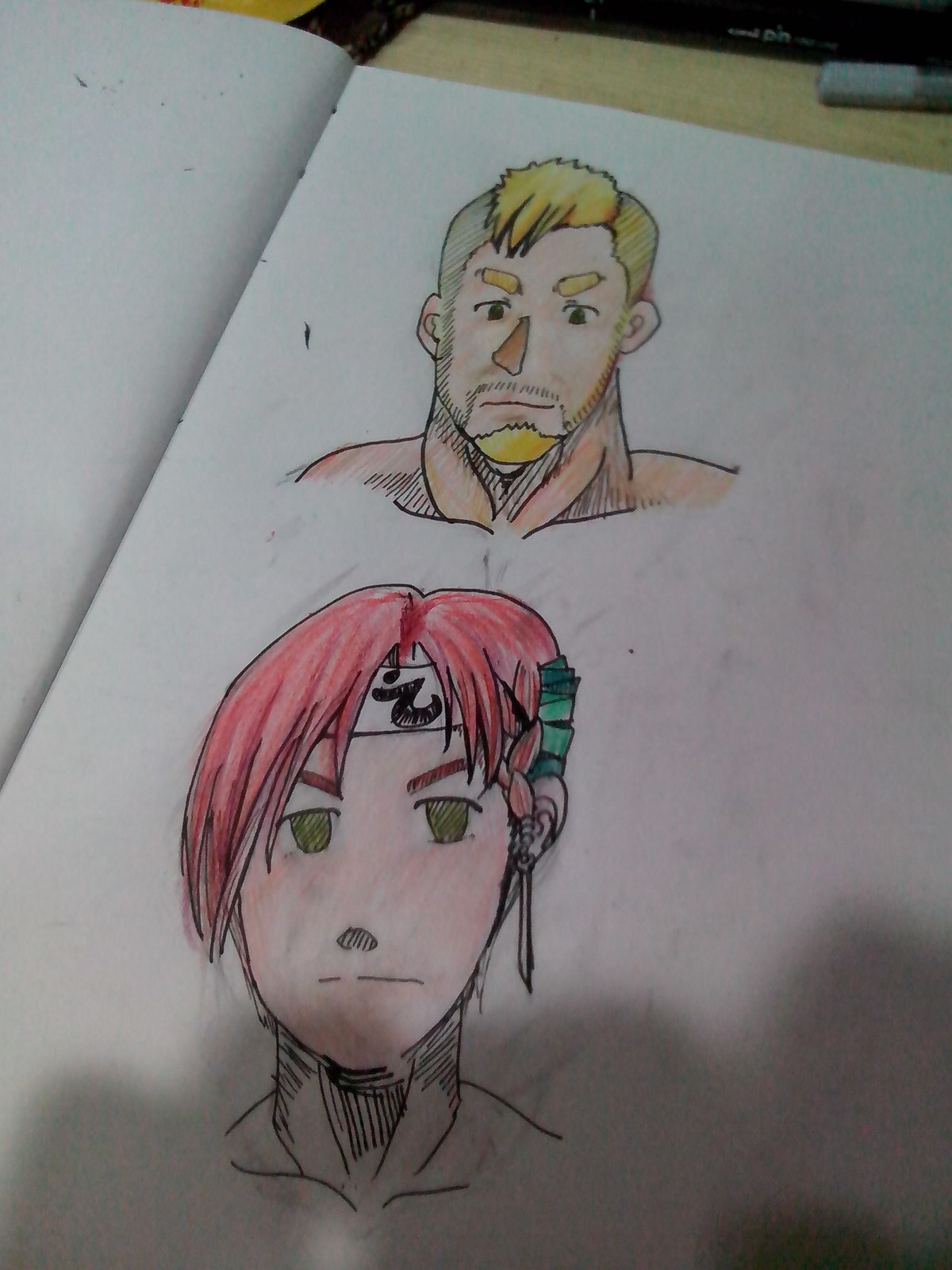The image features two detailed sketches on a white sheet of paper, created using black ink and colored with crayons. The top drawing presents a head and neck portrait of a person with a distinctive blonde Mohawk hairstyle. This individual also sports matching blonde eyebrows and a mustache, complemented by piercing black eyes and a thick muscular neck, which enhances the robust appearance. Below is a second drawing of a red-headed young man, depicted with a white headband and an earring resembling a paintbrush. Both portraits are characterized by their vivid and meticulous detailing, capturing unique and expressive features.